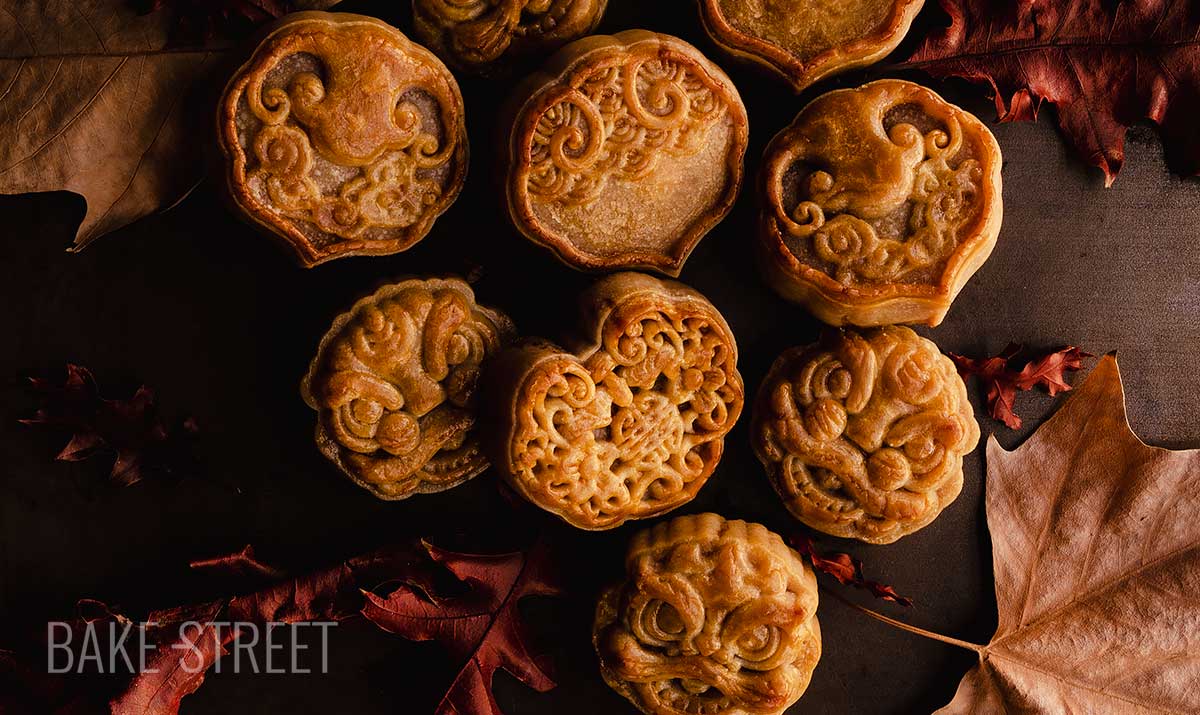In the image, there is a beautifully arranged display of intricately designed mooncakes, typically associated with Asian cultural celebrations like the Lunar New Year. Positioned on a rustic, brown wooden table or possibly atop a tablecloth, the mooncakes are meticulously organized into two rows of three, with an additional lone mooncake situated beneath the middle of the bottom row, creating a visually appealing column effect. The mooncakes feature elaborate patterns, including three that showcase detailed Chinese dragon faces commonly seen in New Year festivities, skillfully crafted from the dough. The other mooncakes bear elegant, swirling designs reminiscent of delicate lotus leaves or traditional Asian crests, with intricate interconnecting lines and ornamental curls.

The scene is decorated with scattered autumn leaves, comprising a mix of vibrant red and earthy brown hues, likely from oak and maple trees, enhancing the seasonal, fall atmosphere of the picture. The lighting highlights the mooncakes, casting the surrounding area in a subtle shadow, reinforcing the autumnal theme. In the bottom left corner of the image, the text "Bake Street" appears in white, with a hyphen-like separator between "Bake" and "Street," adding a professional touch indicative of an advertisement or promotional material.